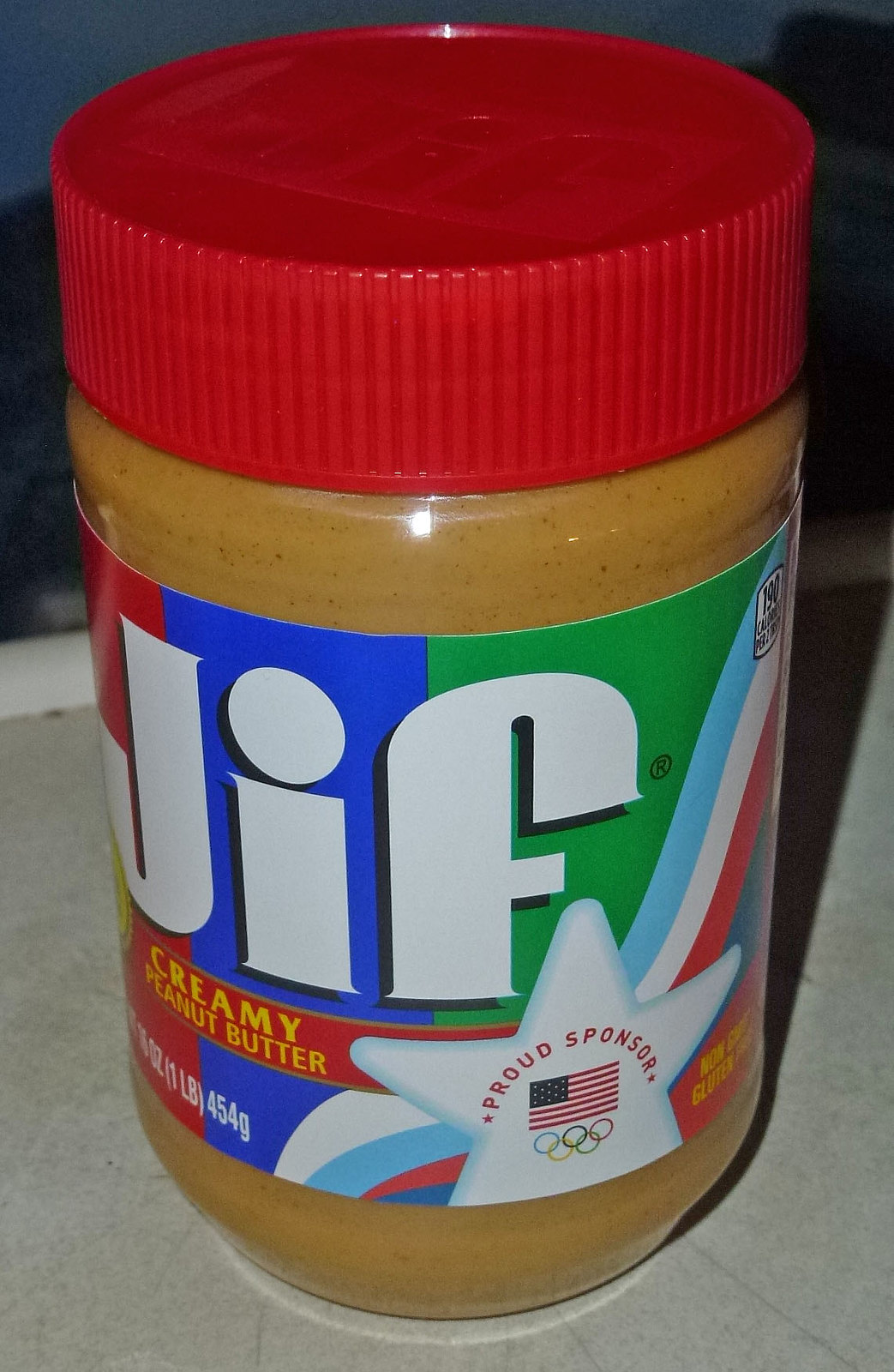This is a detailed photograph of a cylindrical plastic jar of Jif creamy peanut butter, taken indoors on a table with a gray surface and a white border. The jar is clear, showcasing the rich brown peanut butter inside, and is topped with a circular red ridged cap, which has the word "Jif" imprinted on it. The jar is adorned with a tri-colored label featuring red, blue, and green stripes, with the brand name "Jif" prominently displayed in bold white letters. Below the brand name, in a red rectangle, the text "creamy peanut butter" is written in yellow. Additionally, a white star logo with the text "Proud Sponsor," the American flag, and the Olympic rings symbol are displayed, indicating the brand's sponsorship. The label also includes the weight of the product, marked as "16 OZ (1 LB) 454 G." The overall lighting in the photograph highlights the product well, despite the upper part of the image being predominantly dark.